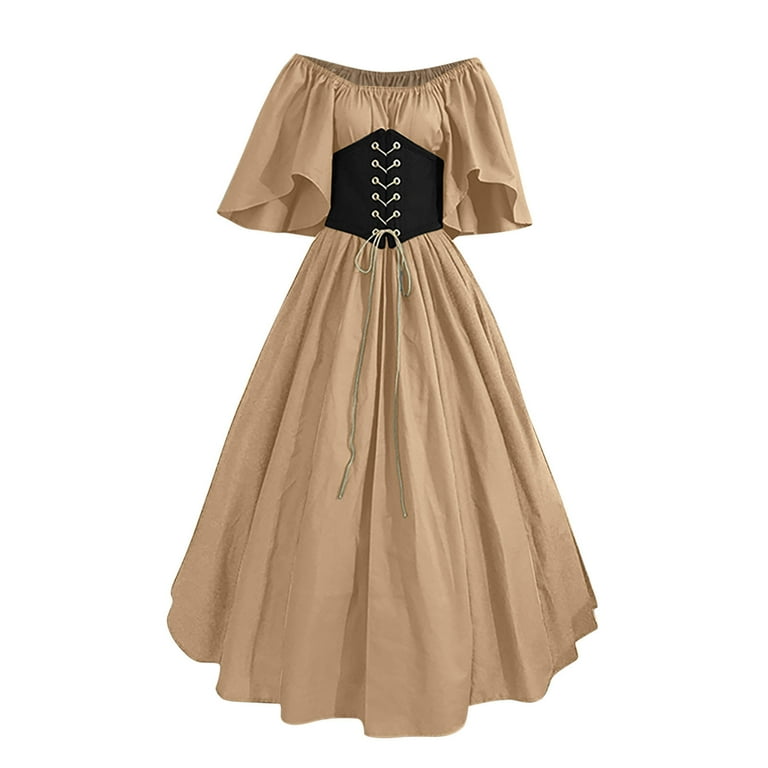The image showcases a vintage, medieval-inspired dress set against a stark white background, giving it an isolated, product-focused appearance. The dress itself is of a light tan, almost cream color, and is designed to be off-shoulder with loose, flowing sleeves that reach just above the elbows. It features a long, pleated skirt that falls to just above the ankle in an A-line shape, reminiscent of historical or pirate era attire. A prominent black corset cinches the waist, made of flat material and threaded with dull white laces that can be adjusted for tightness. The dress, laid out as if worn but with no body inside it, gives a clear view of its structure and elegant details.